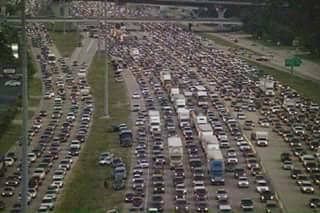An aerial photograph captures a congested highway scene, likely in China due to the unusual twelve-lane configuration not commonly found in the United States. The image shows a stark contrast between a four-lane highway on the left and a massive twelve-lane highway on the right, separated by a grassy divider. On the right side, vehicles are moving forward, heavily populated with numerous white trucks interspersed among multicolored cars, predominantly darker hues. On the left side, cars are driving in the opposite direction, away from the viewer, with noticeably fewer trucks. Some vehicles have spilled over onto the grassy shoulder, adding to the chaotic sense of congestion.